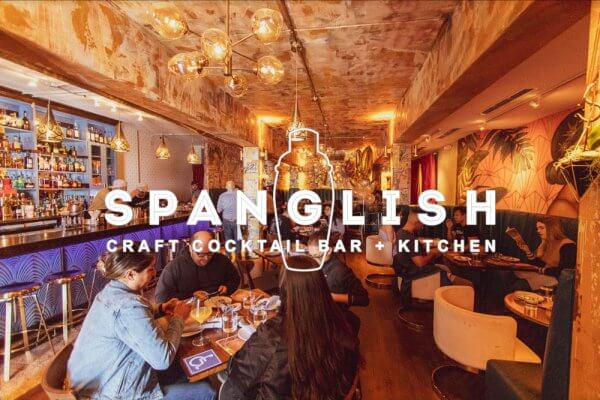The image depicts the interior of a modern, hipster-style restaurant and bar named Spanglish. The setting features a low wooden ceiling with a large lamp hanging down, comprised of six distinct round bulbs. Dominating the center of the image is substantial white text reading "Spanglish," framed by the outline of a cocktail shaker, and below it, the tagline "Craft Cocktail Bar Plus Kitchen." This text partially obscures a group of patrons seated at a table. To the right, a series of large curved white chairs are positioned along tables and booths, indicating additional seating areas. The left side of the space features traditional bar seating extending away from the viewer's perspective. Overall, the image effectively showcases the restaurant's trendy and inviting atmosphere.